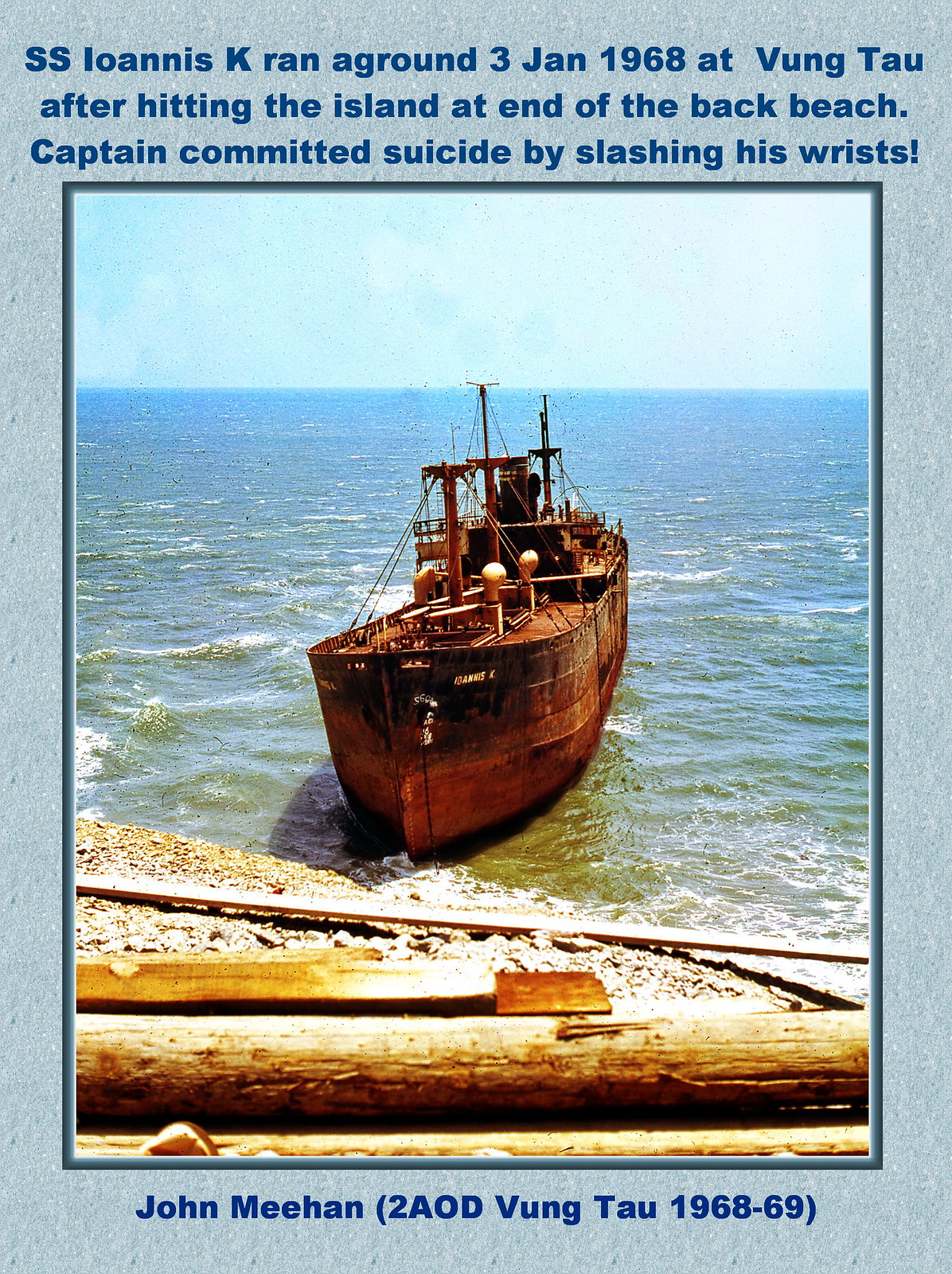The postcard features a historic and tragic image of the SS Loannis K, a freighter that ran aground on January 3rd, 1968, at Vung Tau after striking an island at the end of the back beach. The caption at the top of the postcard notes the unfortunate event of the captain committing suicide by slashing his wrists. Beneath the caption, the name John Meehan is listed, along with “2AOD Vung Tau, 1968 to 1969.” 

In the foreground, the photograph shows the rusted and weathered ship resting against the island's rocky shore. The image is bordered by a light blue frame and includes various earthy and sea tones such as greenish ocean water, brown and orange hues of the rusted ship, and flashes of yellow and gray. The setting appears to be outdoors in the middle of the day, capturing the poignant moment in a bright but somber depiction. Notably, some wooden telephone poles are situated in front of the stranded ship, adding to the scene's historical ambiance.